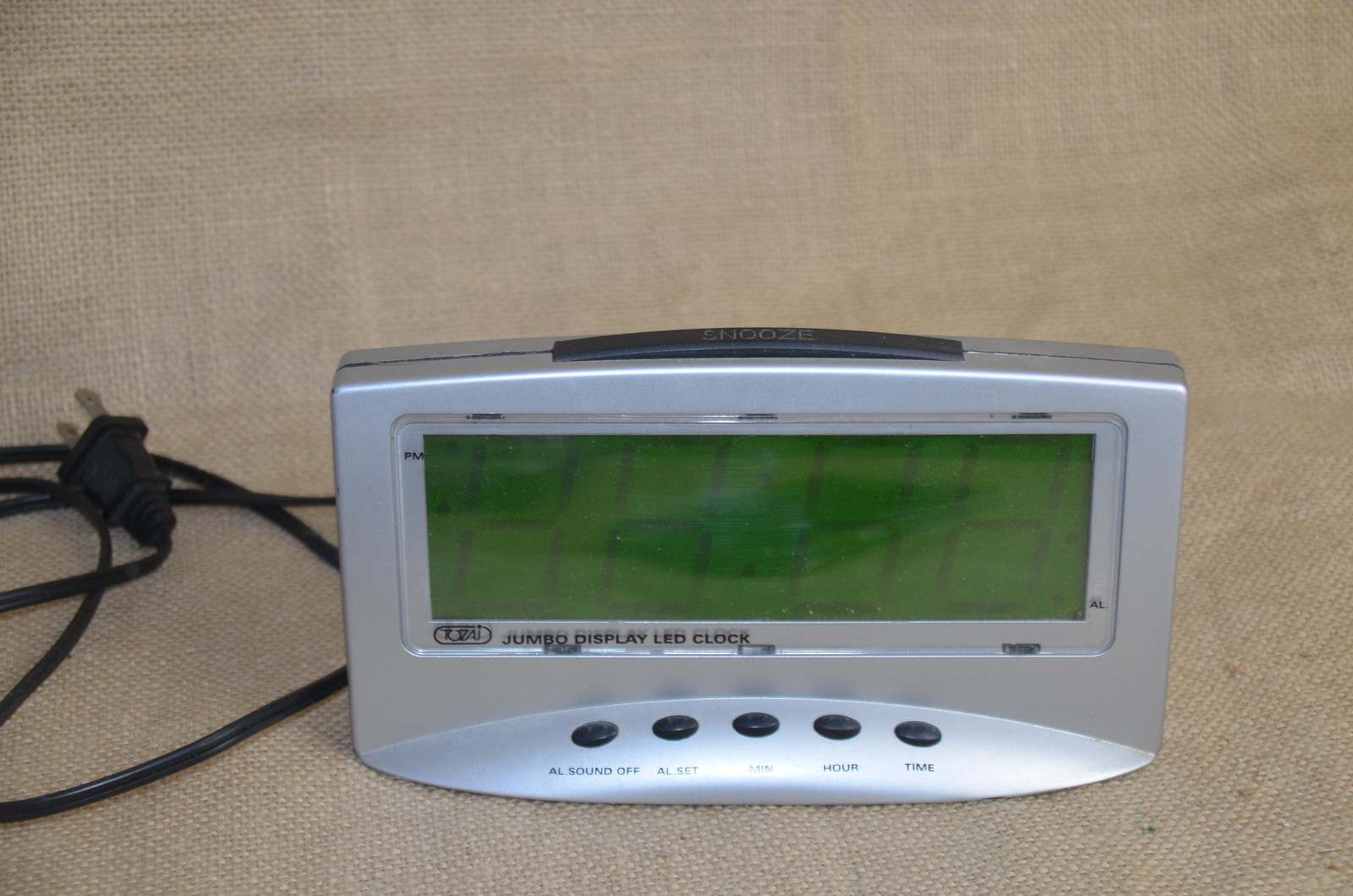This photograph features a modern landscape-oriented electric clock resting on a cream, burlap-textured surface. The clock, designed to resemble a standard bedside table clock, is made of grey plastic. It is currently unplugged, with its black power cord lying nearby. The digital display, inactive due to the clock being unplugged, typically shows dark grey numbers against a light grey background when in use. Positioned on top of the clock is a dark grey snooze button. The clock face includes several control buttons for setting the alarm sound on or off, adjusting the alert times, and other time-related settings. The clock prominently displays "Jumbo Display LED Clock," although the specific brand name underneath is too small to discern.